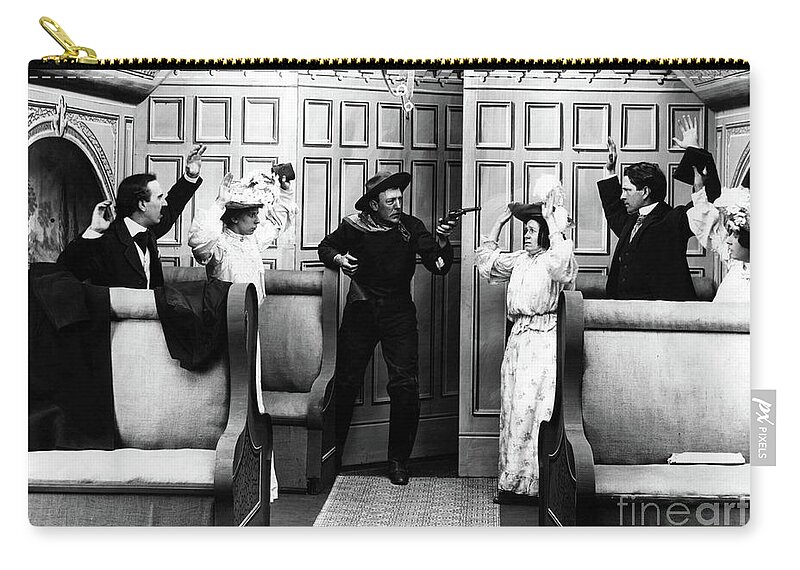This detailed black-and-white photograph, seemingly from the early 20th century, captures a tense moment in what appears to be a train car or similar waiting area with high-backed booth seats. The image is horizontally aligned and prominently features six individuals: three women and three men. The scene is dominated by a middle-aged man dressed entirely in black, sporting a black cowboy hat and brandishing an old-fashioned revolver in his left hand as he gestures menacingly at three of the other people. The remaining five individuals, including three women in elaborate white dresses and large fancy hats, and two men in black suits with early 20th-century hairstyles, have their hands raised in fear. Their expressions, especially the women's, reflect palpable fear. Behind them, a wooden paneled wall and a slightly open door hint at the robber's recent entry. The photo includes a watermark labeled "Fine Art" in the lower right corner and the words "PX Pixels" along the right-hand side. Additionally, the photo appears to be printed on a handbag or similar item, as evidenced by the small gold zipper visible at the top of the image.